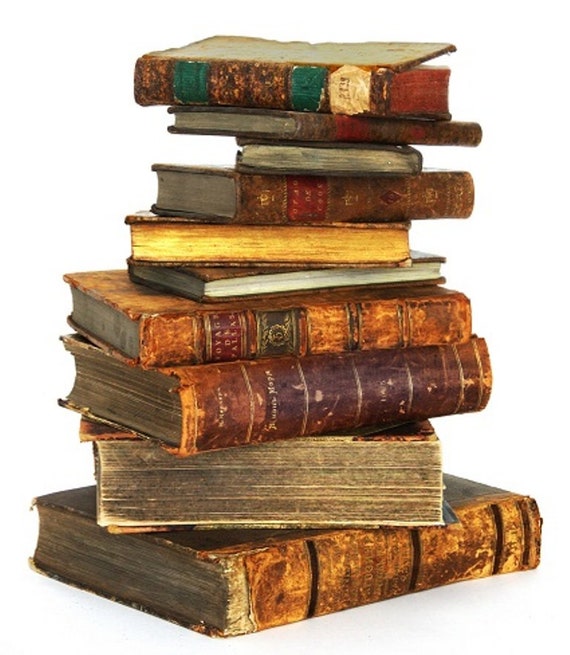A stack of weathered, old books arranged like a sandwich. The largest book at the bottom is oriented towards the right, its tattered cover bearing the marks of age. Above it, a book with its yellowed pages facing the viewer follows. The next two books display their timeworn bindings, aligned in the same direction. The subsequent books gradually decrease in size and alternate in orientation, with some showing their bindings and others their page edges. The overall effect is a haphazard but intriguing arrangement, each book telling its own story through its worn and weather-beaten appearance.